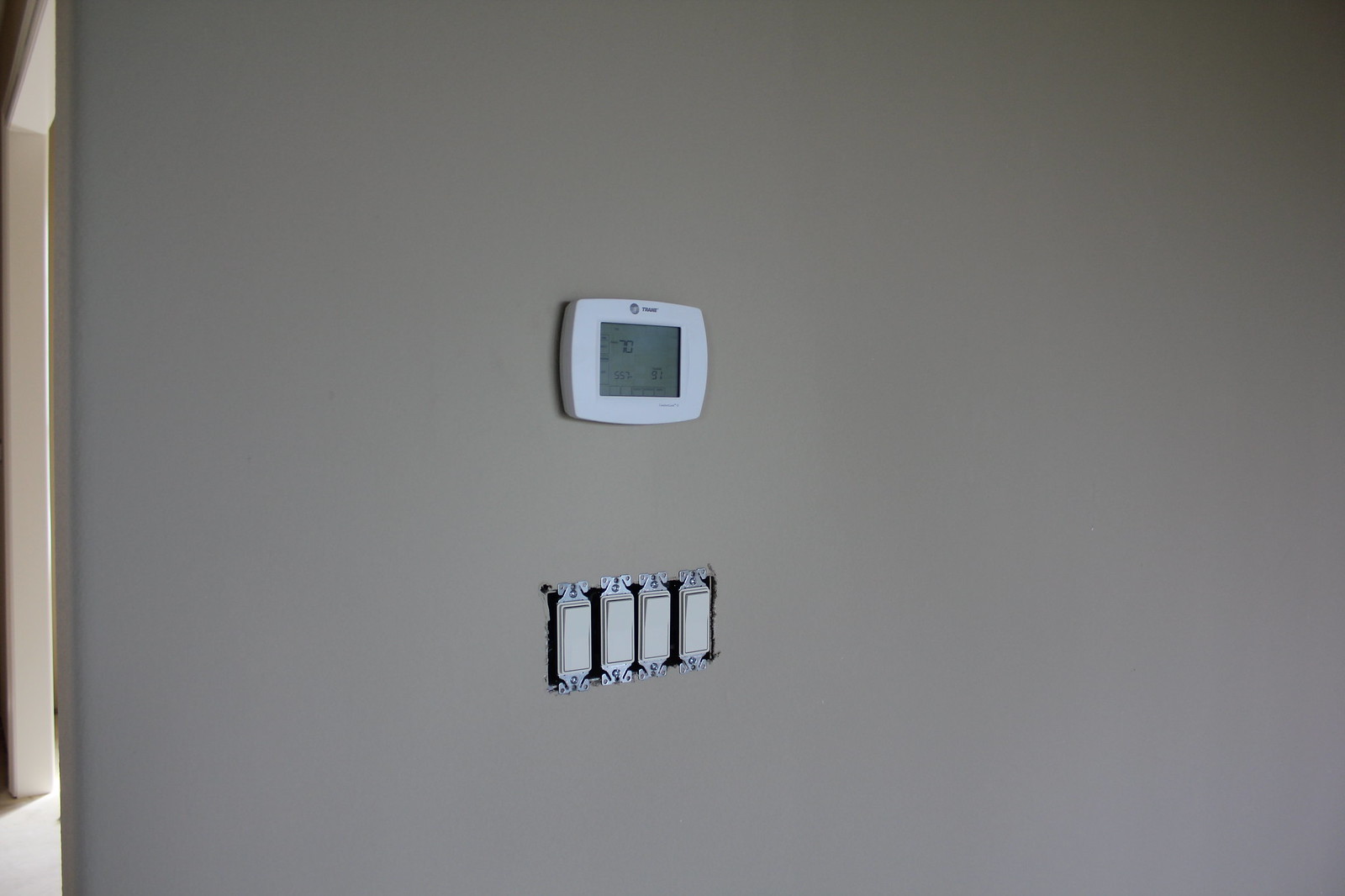The image captures an off-white, nearly gray wall featuring two distinct elements. One element is a rectangular opening outfitted with four vertically aligned, white, raised rectangles, resembling switches. The second element is a white square device with a screen in the center and a logo at the top. The screen displays the number "70" along with other numbers and markings. On the left side of the image, part of an adjacent room's entryway is visible, marked by a long, white column that likely serves as a doorframe. A source of light is emanating from beneath this structure, suggesting illumination from the next room.